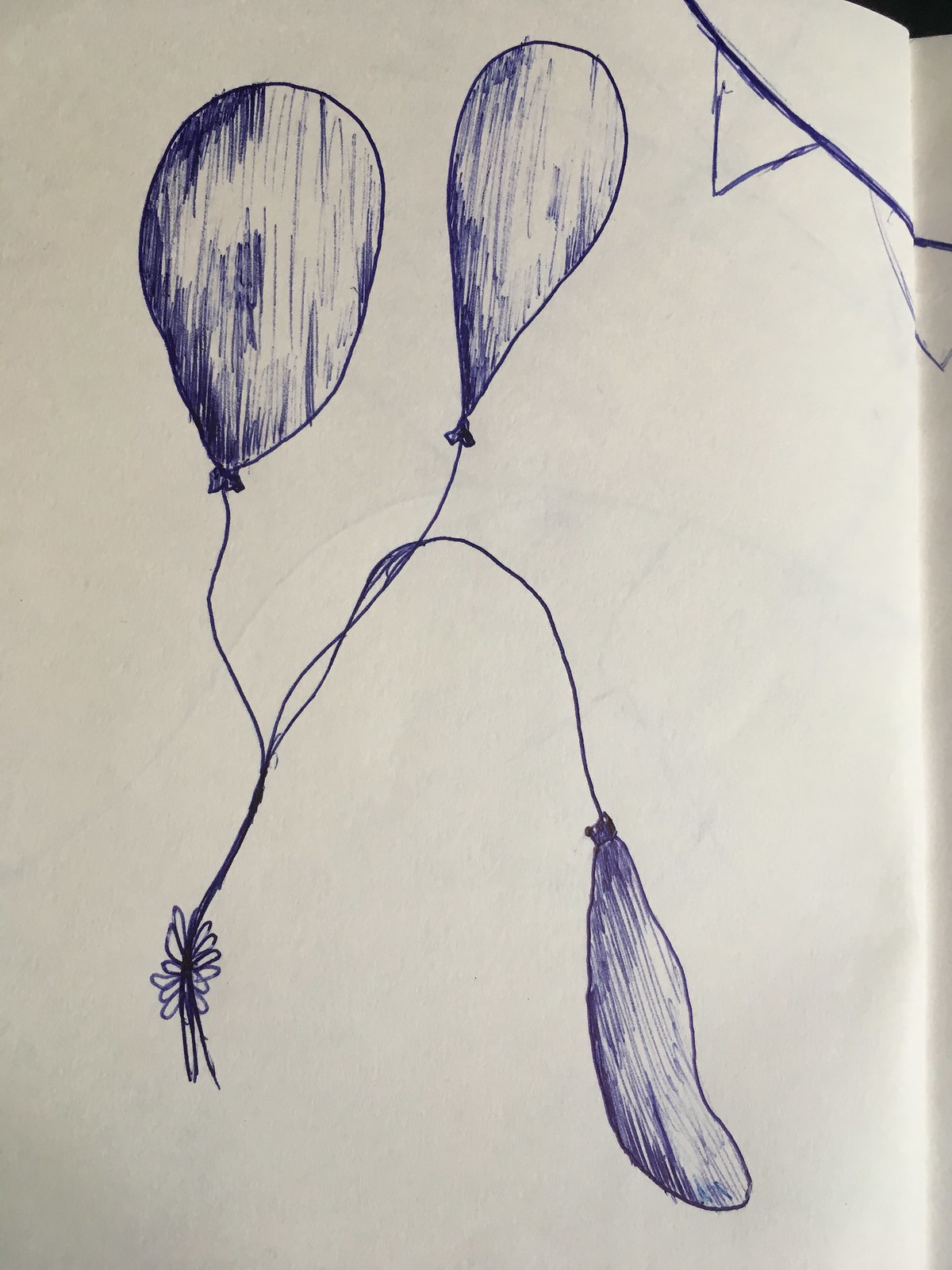The image is a hand-drawn illustration on a blank white piece of paper, created using a blue pen. It features three balloons, each intricately tied at the bottom with a string that forms a flower-like shape. Two of the balloons are depicted floating in the air, one of which is larger than the other. The third balloon appears deflated or in the process of deflating, illustrated as falling. In the top right corner, there are two visible triangular shapes that resemble flags or a banner, evoking a festive atmosphere similar to what one might see at a party.